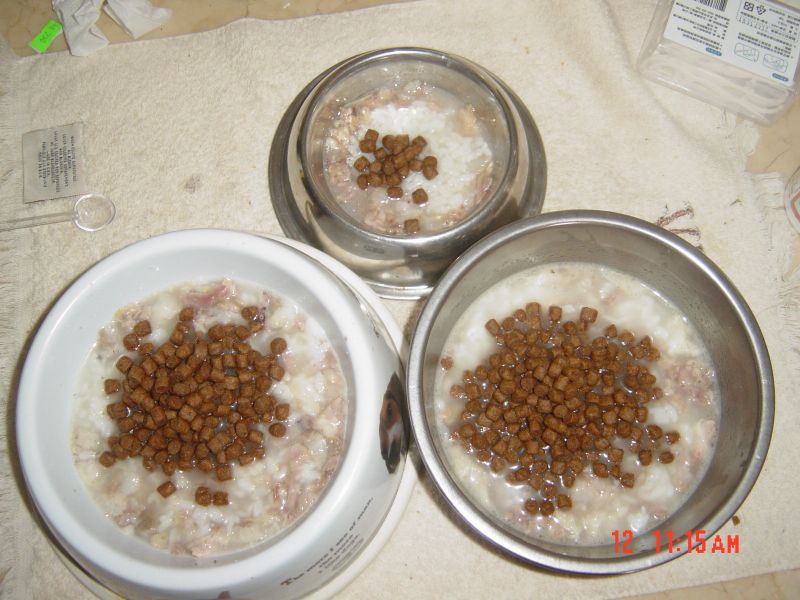The image showcases three dog bowls arranged on a white, slightly yellow-stained cloth. The two larger, round metal bowls feature a mixture of brown and cream kibble along with chunks of meat in a whitish gravy. The smaller, white plastic bowl, adorned with an image of a small dog, holds a similar combination of dog food. Positioned to the far right of the scene, a red digital time display reads 12:11-15 a.m. At the top of the image, a white plastic container and a lime green price label are noticeable. Just above the white bowl on the left, there's a transparent plastic spoon next to a square tag with text, suggesting it might describe the contents of the fabric beneath the bowls.